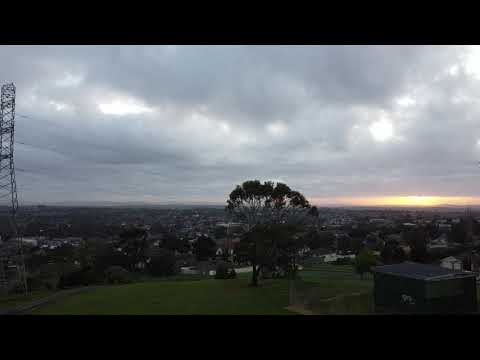This image captures a serene, albeit somewhat dramatic, outdoor scene dominated by a cloudy sky and a vast, green field. The sky, constituting the top half of the picture, is painted in various shades of gray with a hint of yellow and orange hues on the bottom right, suggesting a setting sun. Centered within the lower half of the image are two large, dark trees standing prominently in the lush green grass. To the left side, a towering metal power line structure intrudes into the landscape, leading wires across the overcast backdrop. In the distance, a suburban town sprawls with indistinct buildings and houses interspersed with more greenery, fading into the horizon. At the lower right corner of the foreground lies a nondescript, gray structure, possibly a building, adding a subtle urban element to the rustic charm. The overall composition suggests the photo was taken from a high vantage point, perhaps a park overlooking the town, capturing the tranquil yet somewhat somber atmosphere of the setting sun behind dark, sprawling clouds.